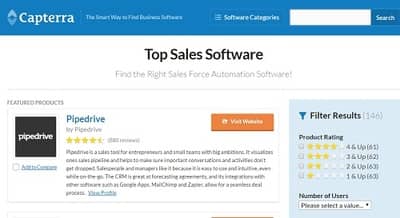This image features a screenshot of the Capterra website displayed on a computer screen. At the top, there's a prominent blue navigation bar stretching across the entire width. On the left side of this bar, a logo is visible comprising two light blue V shapes—one pointing upwards and the other downwards. Adjacent to the logo, the company name "Capterra" is written in white text. Nearby, there are additional white text elements, though these are too small to discern clearly. Further to the right, the words "Software Categories" are accompanied by a three-line icon indicating a drop-down menu. On the far right end of the bar, there's a white search box with a dark blue search button featuring white lettering that reads "Search."

Below this blue bar, the background of the page is primarily white. Centrally positioned in black text are the words "Top Sales Software. Find the right sales force automation software." The first software listed under this heading is "Pipedrive." On the left side of the listing, there's an image of the Pipedrive logo—a black square with the word "Pipedrive" in white text at its center. The listing includes the name of the company behind the software and a brief summary describing its functionalities. To the right of the summary, there's an orange button that allows users to visit the Pipedrive website.

On the far right side of the webpage, there's a blue sidebar with light blue text that reads "Filter Results." This section offers options to filter the software listings based on product rating and the number of users.